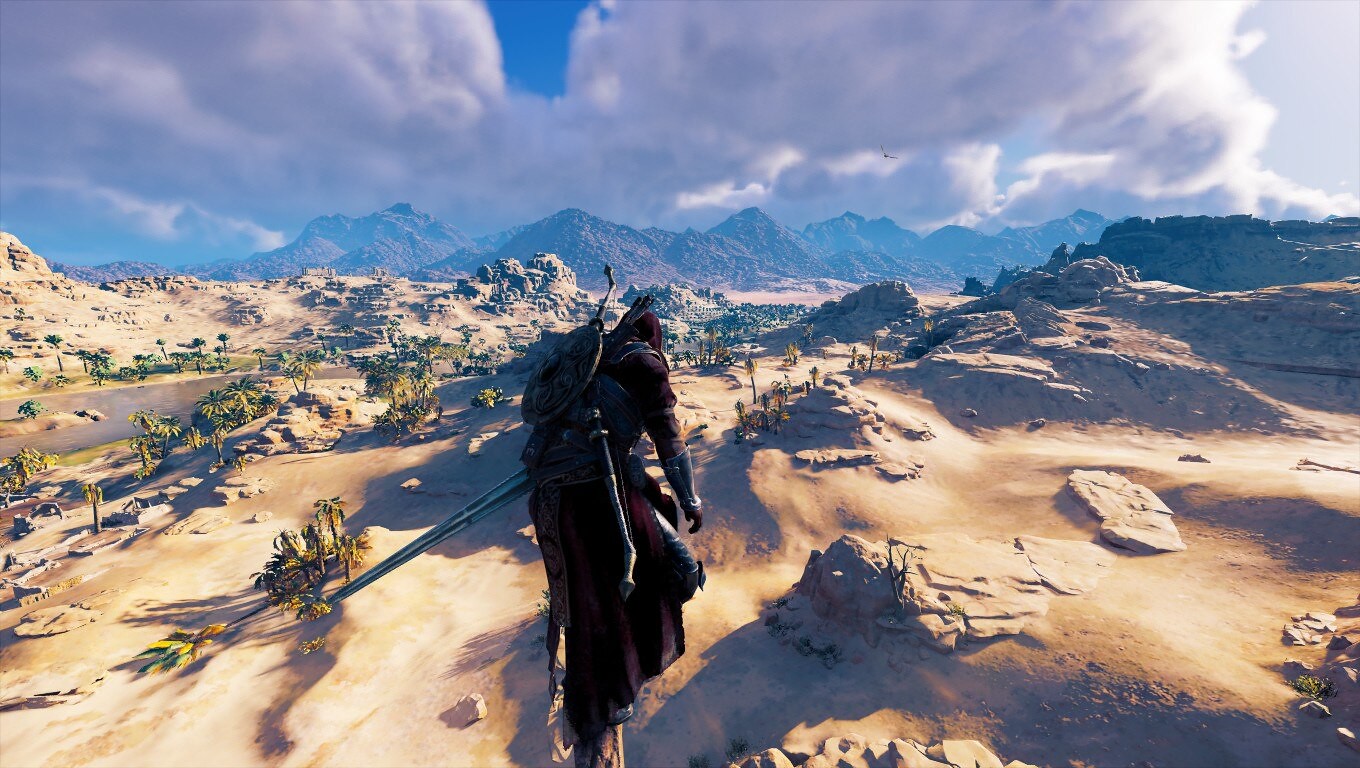In this still image taken from a video game reminiscent of Assassin's Creed, we see an expansive, arid desert landscape characterized by sand dunes, tan-colored rocky formations, and scattered palm trees growing along a thin stream on the left. In the far distance, rugged mountains rise against a blue sky adorned with large, puffy clouds. The video game character, viewed from behind, stands perched on a protruding rock formation, surveying the dry terrain. Clad in a dark crimson or burgundy assassin's robe with a hood that covers their head, the character's attire includes metal gauntlets and a long cloak that reaches the ground. A shield and bow are strapped to their back, while a short sword hangs in a scabbard at their side. The character may be holding a longer sword or has it secured to their left side. All visible parts of their body are fully covered, enhancing their enigmatic presence in this detailed, desolate scenery.